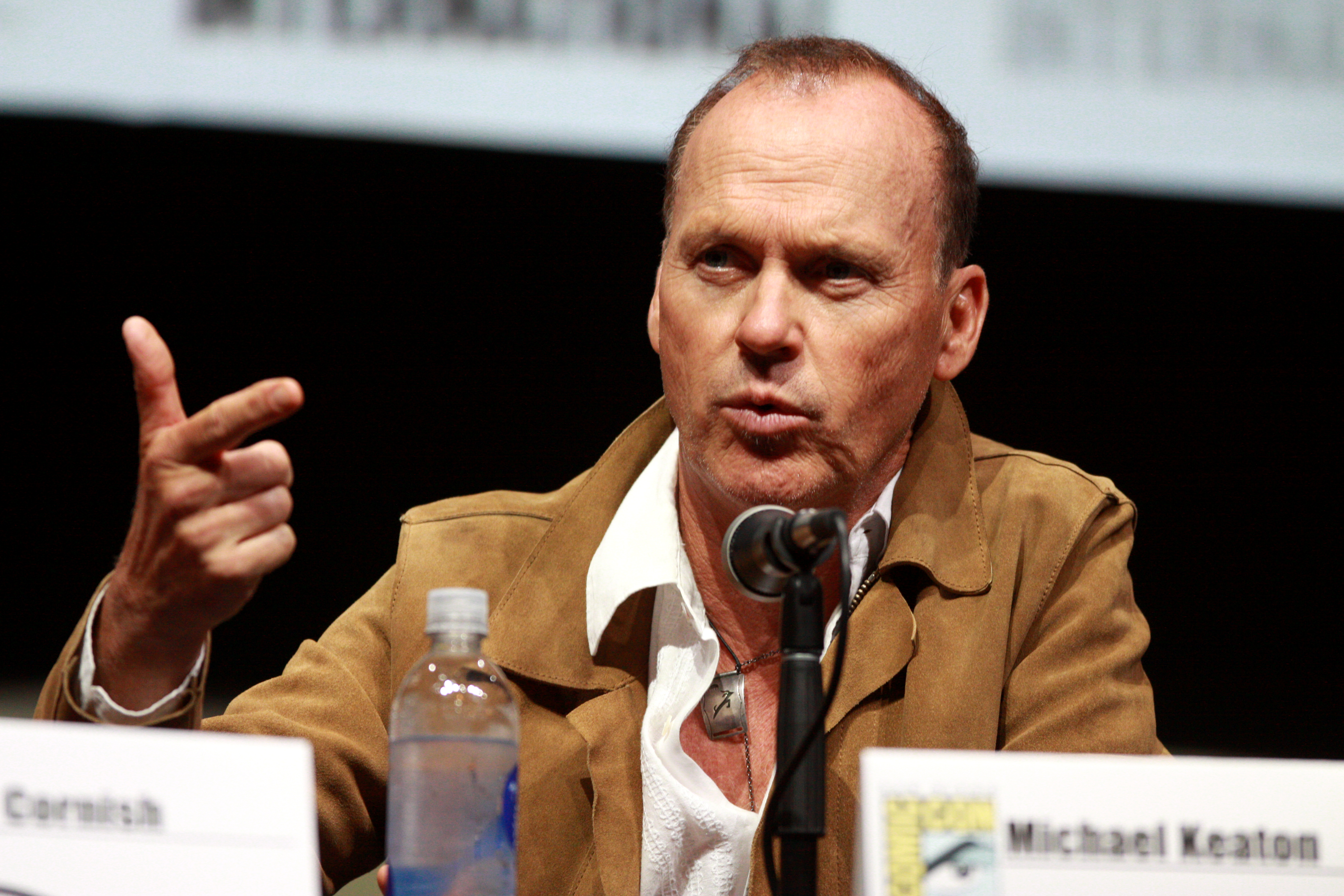This detailed photograph captures a Comic-Con event with actor Michael Keaton at the center. Seated behind a table, Keaton is engaged in speaking at a press meet, with his right hand raised and fingers pointed forward, gesturing as he talks into a black microphone with a silver head. He is dressed in a white shirt and a brown (or khaki) blazer and is wearing a small metal chain around his neck. In front of him, there's a name board displaying "Michael Keaton" alongside the Comic-Con logo, partially blurred but still identifiable. To the left of the microphone sits a plastic water bottle. The table also features a second, less legible name board for another individual seated next to Keaton. The background of the image is blurred, featuring a black and white banner with a white stripe on top.